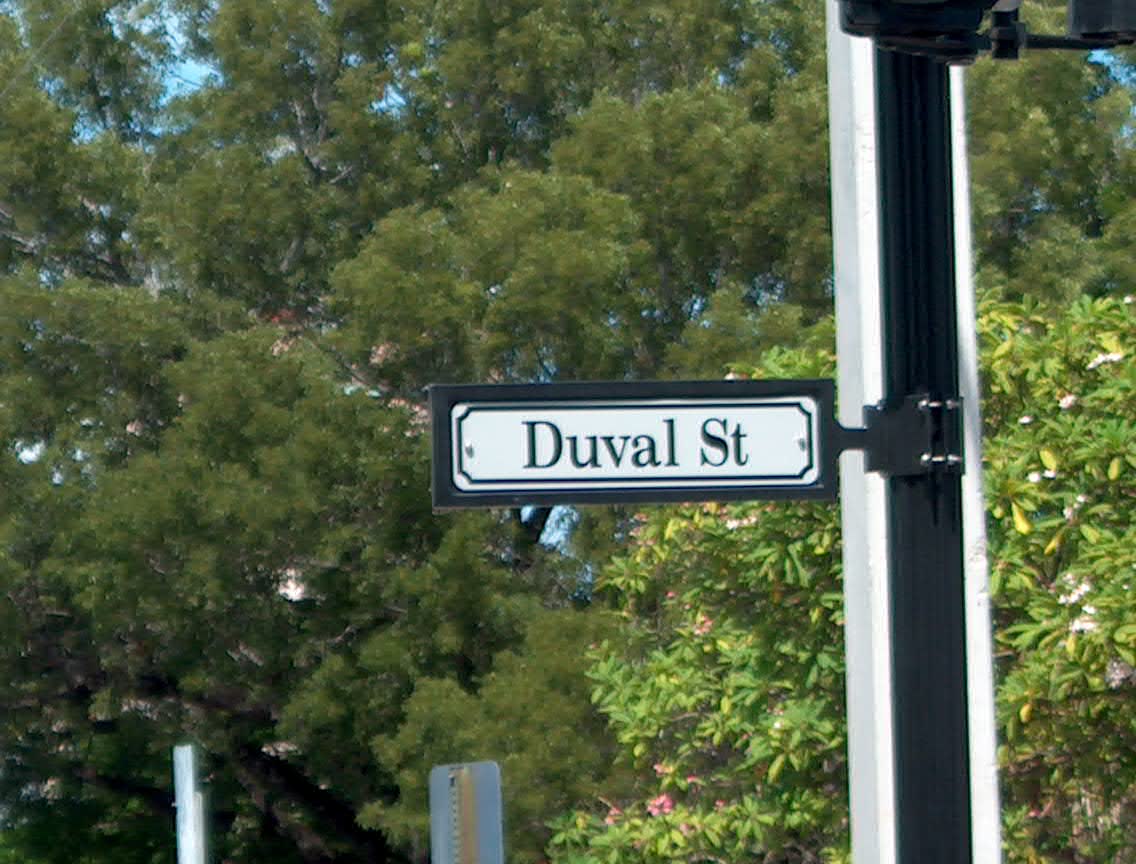This image showcases a Duval Street sign mounted on a notably thick pole situated on the right side of the frame. The pole features a black center flanked by white segments on both sides. The sign itself is black and white, affixed to the pole using two metal brackets bolted together. The Duval Street sign displays bold black letters on a white background. Below this sign, a smaller rectangular sign's back is visible. To the left of the pole are additional posts. On the right, a bush adorned with numerous small purple blossoms is visible, while on the left, lush green trees dominate the scene, obscuring the skylight above.